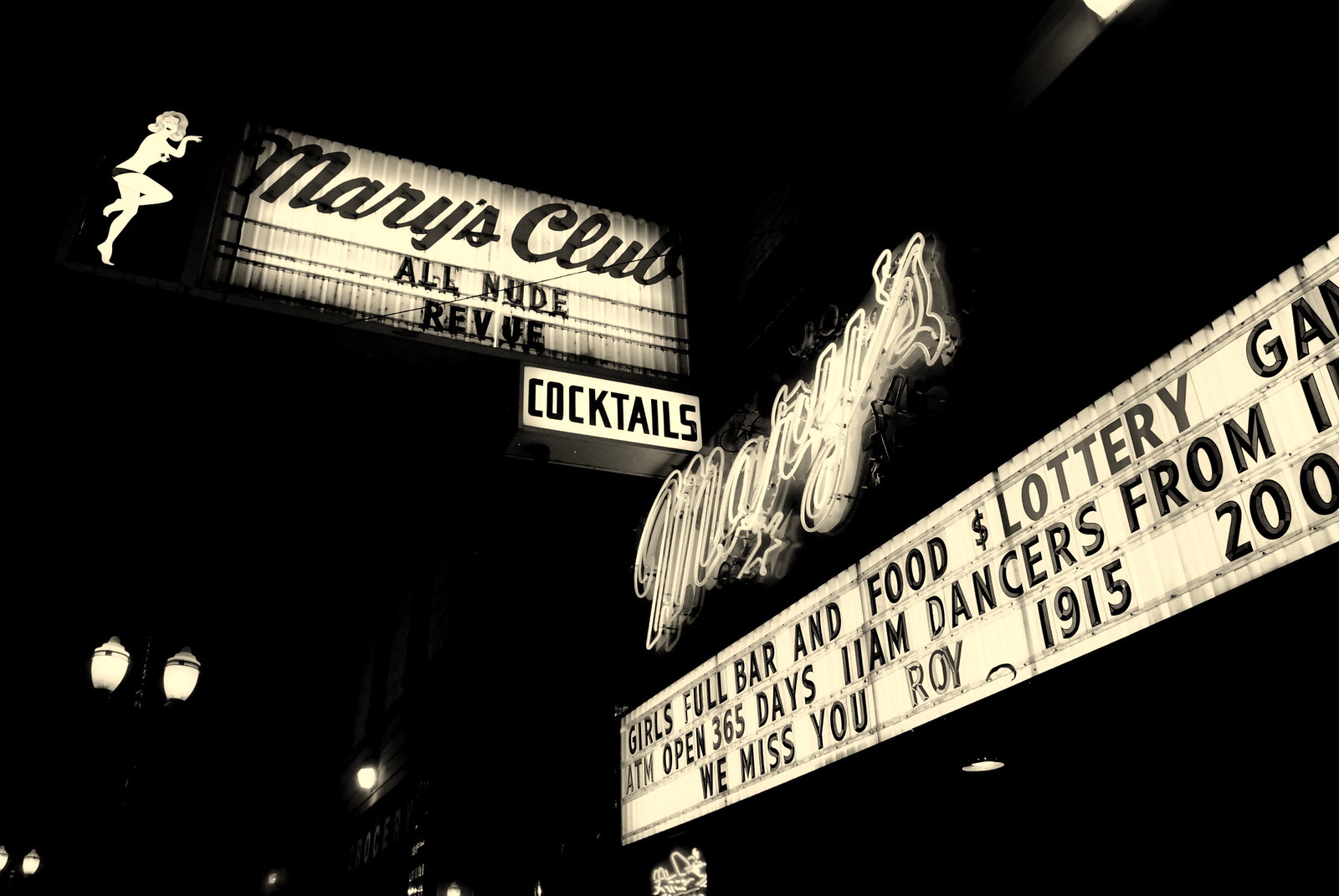This photograph, likely in black and white, captures the exterior of a business at night, illuminated mainly by neon signs and street lamps. In the lower left corner, a couple of street lamps light up the scene, but the real focus is on the brightly lit signage of a building that's largely obscured by darkness. The most prominent feature is a perpendicular sign at the top, showcasing a neon-lit, scantily clad woman next to the text "Mary's Club All Nude Review." Just beneath, the sign reads "Cocktails." Further down on the building, a cursive neon sign displays "Mary's" with a star underneath. Below this, another sign features changeable letters spelling out "Girls Full Bar and Food Lottery ATM open 365 days 11 a.m. Dancers from We Miss You Roy 1915 to 2000 something." The right side of this lower sign is cut off, adding to the enigmatic atmosphere of the scene.